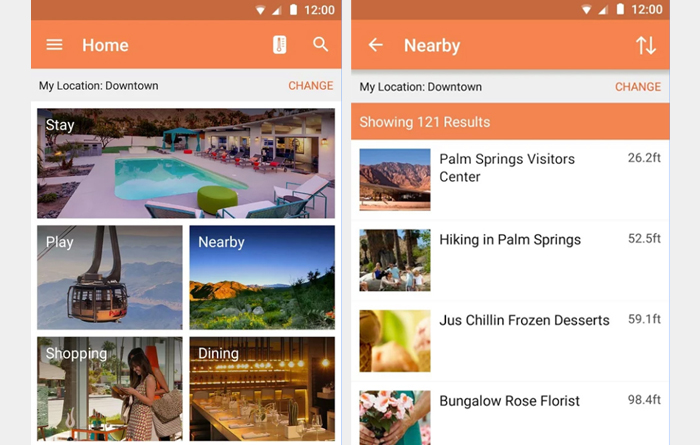Two side-by-side screenshots from a phone display information about downtown locations. The top portion of each screenshot is highlighted in orange, while the remainder of the content is set against a white background.

In the first screenshot, the heading reads "My Location: Downtown," beneath which are categories labeled "Stay," "Play," "Nearby," "Shopping," and "Dining." Accompanying images include a hotel for "Stay," a ski lift for "Play," scenic mountains for "Nearby," a woman shopping for "Shopping," and an upscale restaurant for "Dining." The text also mentions "121 results."

The second screenshot provides specific recommendations within close proximity: the Palm Springs Visitor Center located just 26.2 feet away, a hiking spot in Palm Springs at 52.5 feet, Just Chillin' Frozen Desserts at 59.1 feet, and Bungalow Rose Florist at 98.4 feet.